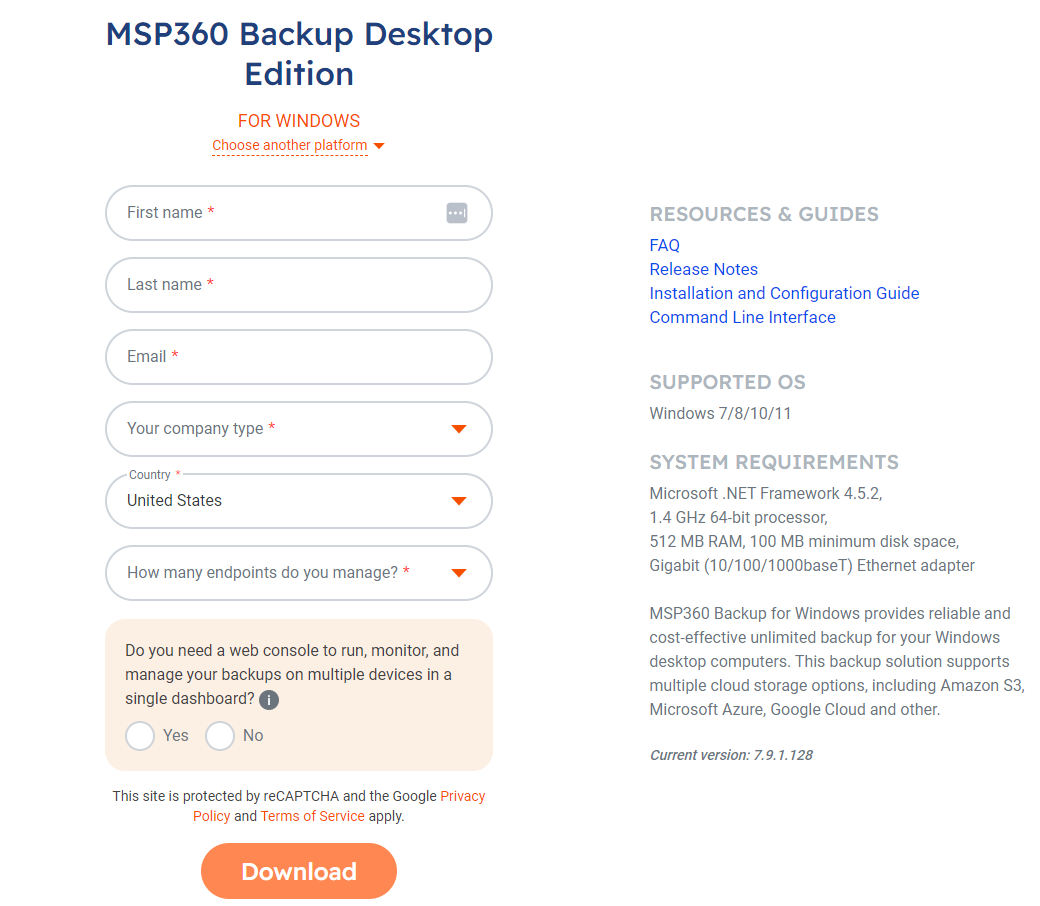The image is a screenshot with a white background, divided into a left and a right section. The left section's header reads "MSP360 Backup Desktop Edition" followed by a subtitle in orange, "For Windows," and a choice to "Choose Another Platform" with a down arrow beside it. Below this header are a series of input fields denoted by bubbles, each allowing for user interaction. These fields prompt for "First Name," "Last Name," "Email," and "Your Company Type" with a drop-down arrow. The country is pre-selected as "United States" with another drop-down arrow, and there is a field for "How Many Endpoints Do You Manage" with a corresponding drop-down arrow.

Further down, a small light orange box inquires, "Do You Need a Web Console to Run, Monitor, and Manage Your Backups on Multiple Devices in a Single Dashboard?" with "Yes" and "No" choice buttons. Beneath this query, a disclaimer states, "This site is protected by reCAPTCHA and the Google Privacy Policy and Terms of Service Apply." An orange "Download" button is prominently displayed at the bottom of the left section.

The right section consists of three main headings: "Resources and Guides," "Supported OS," and "System Requirements." Under "Resources and Guides," four clickable links are provided: "FAQ," "Release Notes," "Installation and Configuration Guide," and "Command Line Interface." The "System Requirements" section lists the necessary prerequisites for using the software. At the bottom of the right column, the current software version is listed as "Current Version 7.9.1.128."